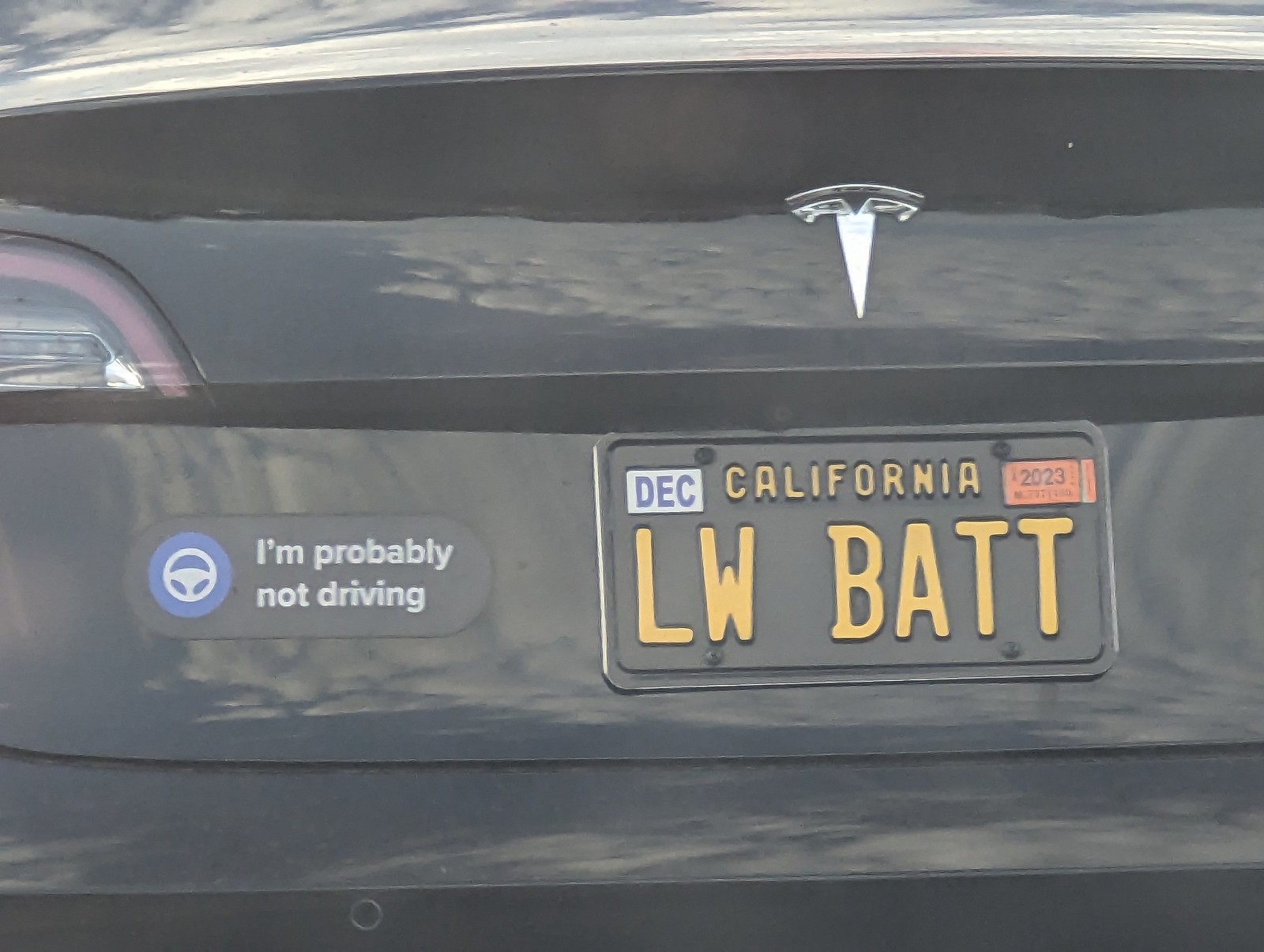This image shows the rear end of a shiny black Tesla automobile, reflecting the sky on its surface. The centerpiece of the photo is the vehicle's personalized California license plate with yellow letters on a black background, displaying "LWBATT." The registration details are visible on the plate, with a white "DEC" sticker in the upper left corner indicating expiration in December, and a red "2023" sticker on the right side. To the left of the license plate, a black bumper sticker with white lettering reads, "I'm probably not driving," underscored by a blue circle with a white steering wheel icon, suggesting the car's autonomous driving capabilities. The Tesla emblem is prominently displayed on the trunk, partially shadowed by the back fin. The taillights, featuring a blend of faded red and clear sections, are mostly visible on the upper left, while the bottom left showcases the circular area housing the backup camera.